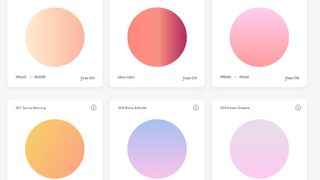This cropped screenshot showcases a detailed color palette arranged in two horizontal rows of three colors each, with each color encapsulated in a small white box. The white boxes are set against a gray background. The labels beneath the colors include shade names on the left and numerical values on the right, though some information is cut off due to the cropping.

In the top row, the first box to the left contains a peach color. The middle box features a gradient red, transitioning smoothly through varying shades of red. The third box displays a gradient pink, shifting from one shade of pink to another.

The bottom row follows a similar structure. The first box on the left presents an orange color. The center box displays a gradient purple, transitioning through different purple tones. The third box on the right shows a gradient light pink, starting with a darker pink at the top and fading into a lighter pink as it reaches the bottom.

Unfortunately, the top edges of the colors in the upper row and the bottom edges of the lower row are cropped out, limiting the complete view of the shades.